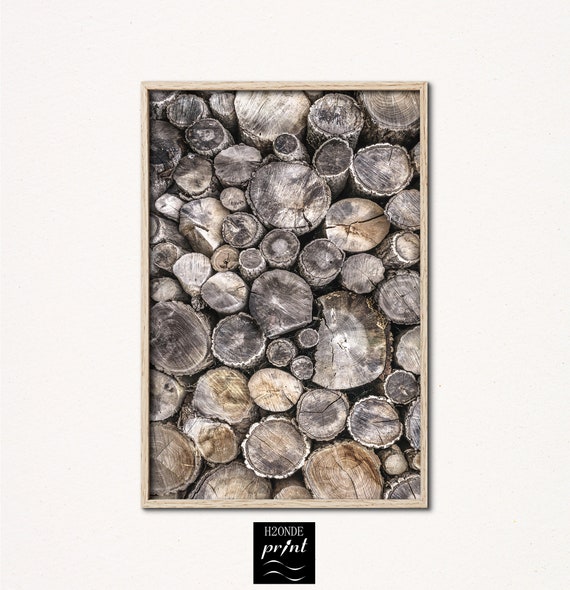The image showcases various pieces of chopped wood, intricately detailed and appearing as an aerial view of stumps in a painting. Each stump is uniquely shaped, ranging from circular to jagged, in colors of brown, teal, white, and gray. The wood pieces are framed in a gray picture frame and set against a plain white background. Below the painting, a black box centrally located at the bottom contains the white text "H20NDEPrint" with two white squiggly lines beneath it, adding a distinctive element to the composition. The knots and details of the wood stumps are vividly captured, contributing to the textured richness of the image.